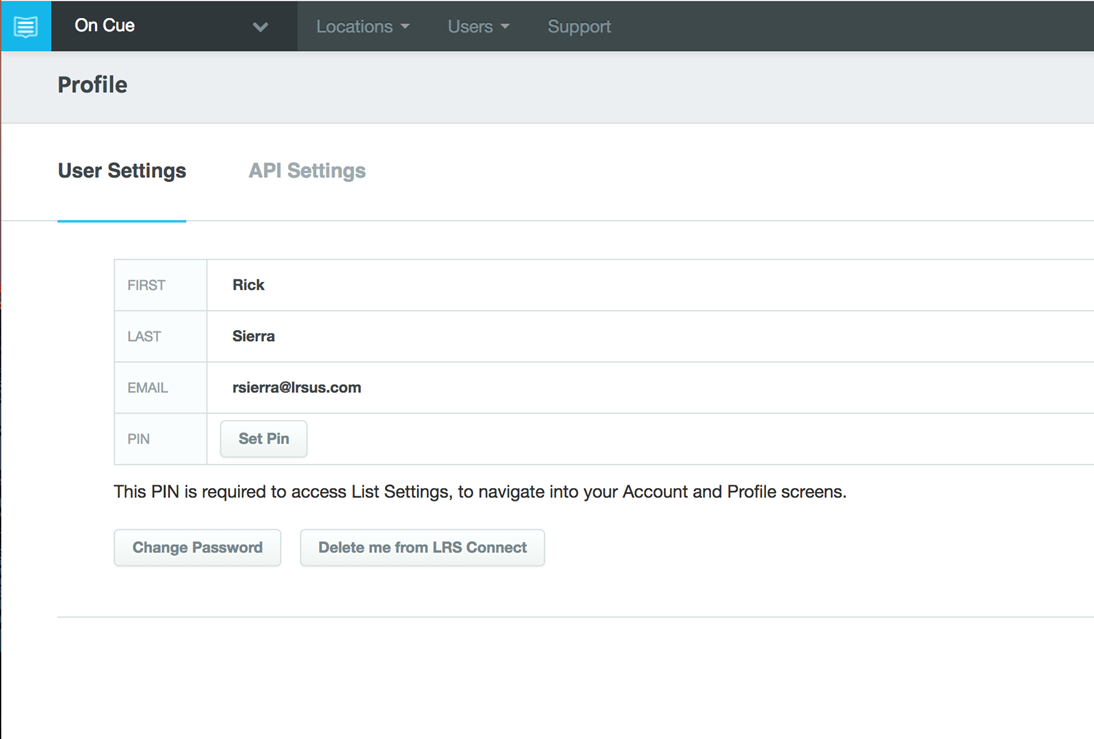This detailed caption describes a cropped screenshot of the OnCue app, which is designed for managing customer paging, waitlists, and table management in the restaurant and hospitality industries. The screenshot displays a user’s profile settings page within the app. At the bottom of the screen, a section labeled "User Settings" can be seen, where fields are provided for entering a first name, last name, and email address. Additionally, there is a gray button labeled "Set PIN," which is described as a necessary step to access list settings and navigate to the account and profile screens. Furthermore, options to "Change Password" and "Delete Me from LRS Connect" appear below. The OnCue app aids in efficient restaurant management, similar to the usage of black table pagers for customer notifications.